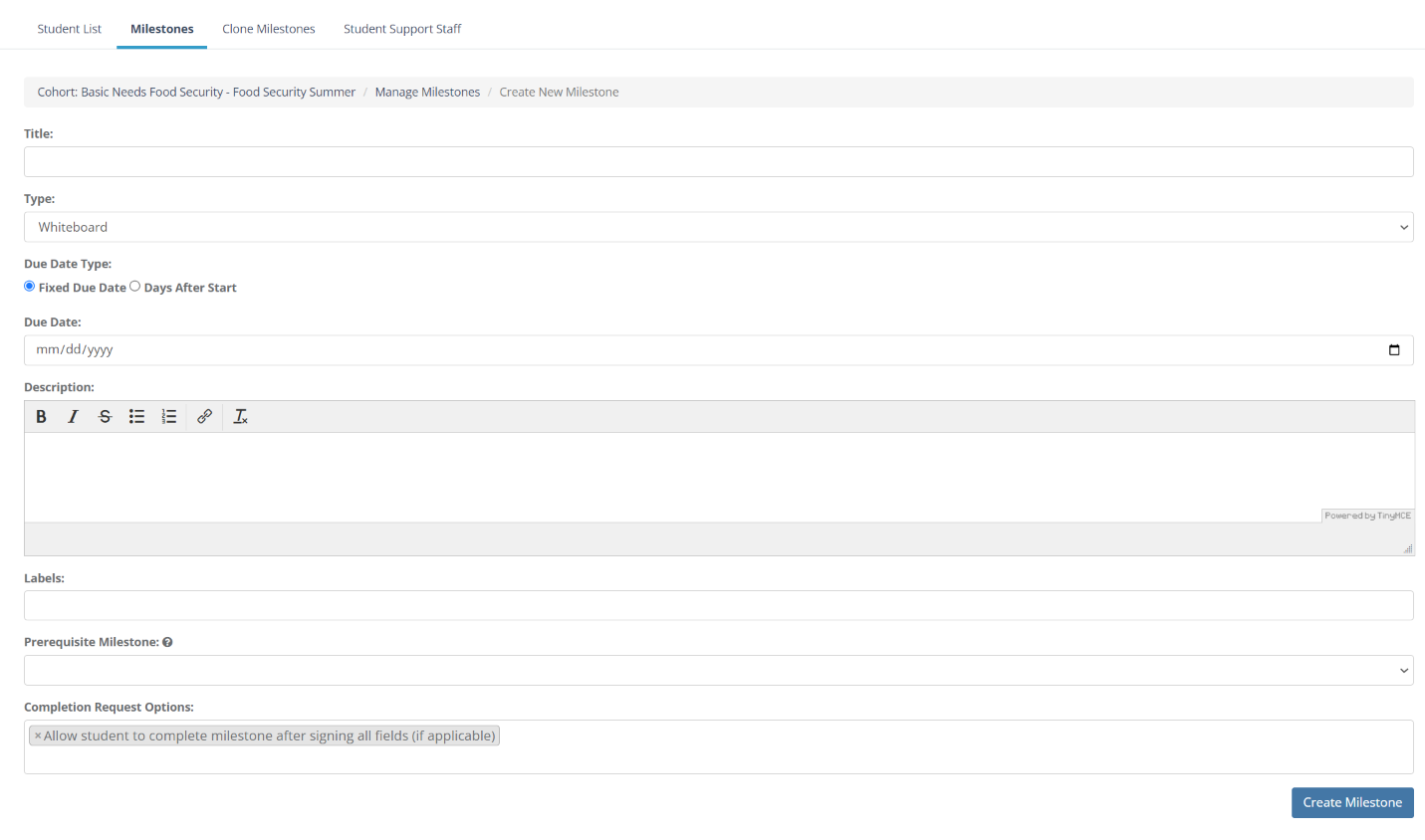This image depicts a screenshot of an interface for managing a student support system. At the top of the page, there are four distinct tabs labeled: "Short List" or "Student List," "Milestones," "Clone Milestones," and "Student Support Staff." Below these tabs, there is a title block that categorizes content under various themes such as "Cohon," "Basic Needs," and "Food Security," with subcategories for "Food Security - Summer" and options to manage or create new milestones.

On the lower part of the page, several information blocks are present. These include sections for defining types of activities (labeled "Whiteboard"), specifying due dates, and categorizing these due dates either as fixed or as a certain number of days after the start of a period. Another area at the bottom features a description box intended for adding detailed explanations or notes. Overall, the layout is designed to streamline the organization and tracking of students' progress and needs.